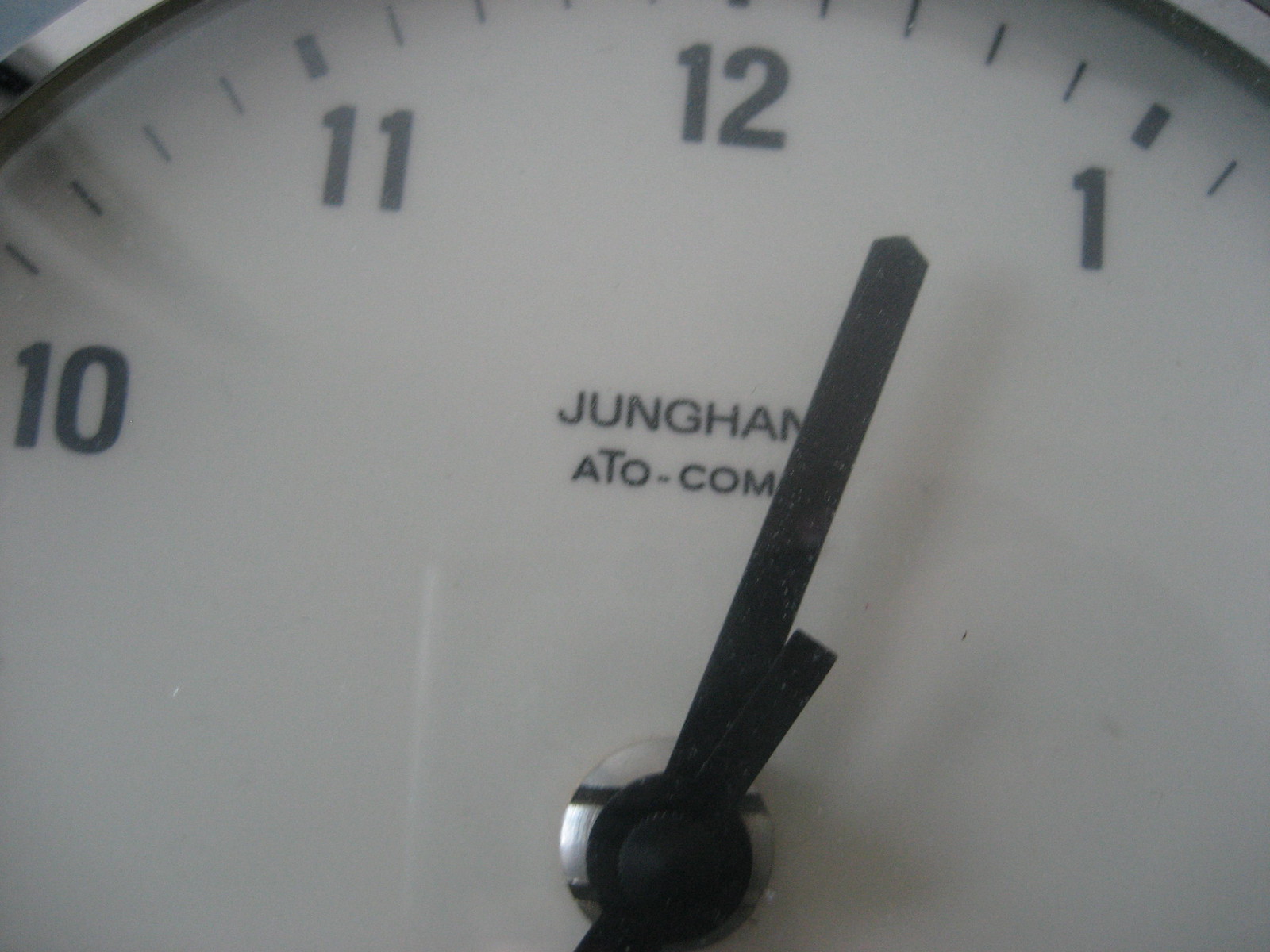The image depicts a close-up view of a wall clock with a silver frame. The clock face prominently displays the numbers 10, 11, 12, and 1, each separated by small black lines that denote the seconds. The hour hand is nearing the 1 o'clock position, while the minute hand's exact position is unclear. The brand name "Junghans" is inscribed on the clock, and beneath it, the text "ATO.COM" is visible.